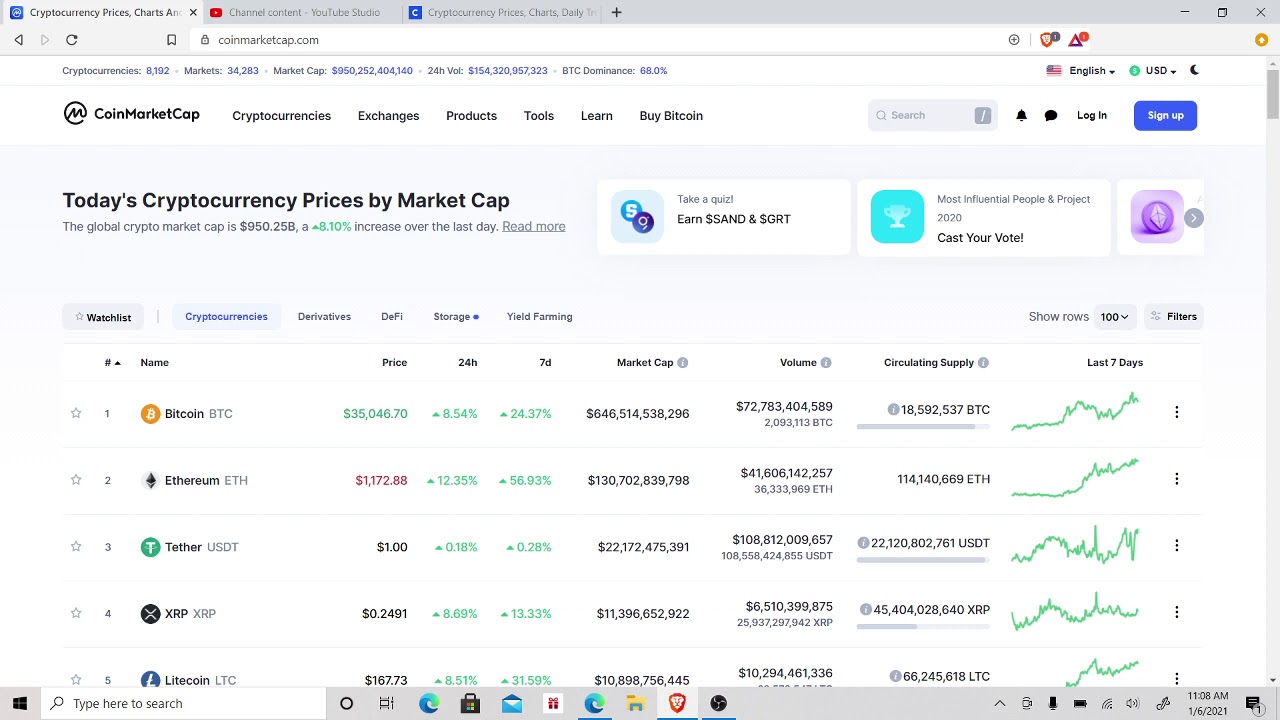This is a detailed, horizontal, left-to-right image depicting a comprehensive cryptocurrency dashboard, resembling what one might encounter on a computer screen. The top of the screen features a gray navigation bar, with the first tab labeled "Cryptocurrency Charts" highlighted as the selected option. Additional tabs include "Channel Content," "YouTube Studio," "Cryptocurrency Prices," "Charts," "Daily," and a plus sign to open a new tab. On the far right of this bar, you find the standard window control buttons: minimize, maximize, and close.

Directly beneath this bar, aligned to the left, are navigation controls including left and right arrows, a refresh icon, a bookmark icon, and a search bar displaying the URL "coinmarketcap.com." Adjacent to these, towards the right, are several additional icons.

Below this section is detailed cryptocurrency information starting with a total count of cryptocurrencies listed as 8,192 followed by various statistics such as the total number of markets, the overall market cap, 24-hour volume, and Bitcoin (BTC) dominance. Language options are available with English (indicated by an American flag) selected, and currency preferences set to USD.

The interface incorporates a moon icon alongside several major navigation options: "Cryptocurrencies," "Exchanges," "Products," "Tools," "Learn," and "Buy Bitcoin." Additional utilities on this row include a search bar, an alarm icon, a messages icon, and buttons for logging in and signing up. On the far right there's a scroll bar for navigating the content.

The main body of the dashboard introduces "Today's Cryptocurrency Prices by Market Cap," alongside interactive elements such as a quiz link, options to view the most influential people and projects of 2020, and a voting mechanism. There’s also mention of a watch list.

A detailed table follows, outlining specifics for various cryptocurrencies, labeled with columns for name, price, 24-hour change, 7-day change, market cap, volume, circulating supply, and performance over the last 7 days. Filtering options are available to refine the displayed data.

The image concludes with the typical computer taskbar at the very bottom, showing various desktop icons. This visually rich and information-dense interface is tailored to deliver a complete real-time cryptocurrency market analysis.